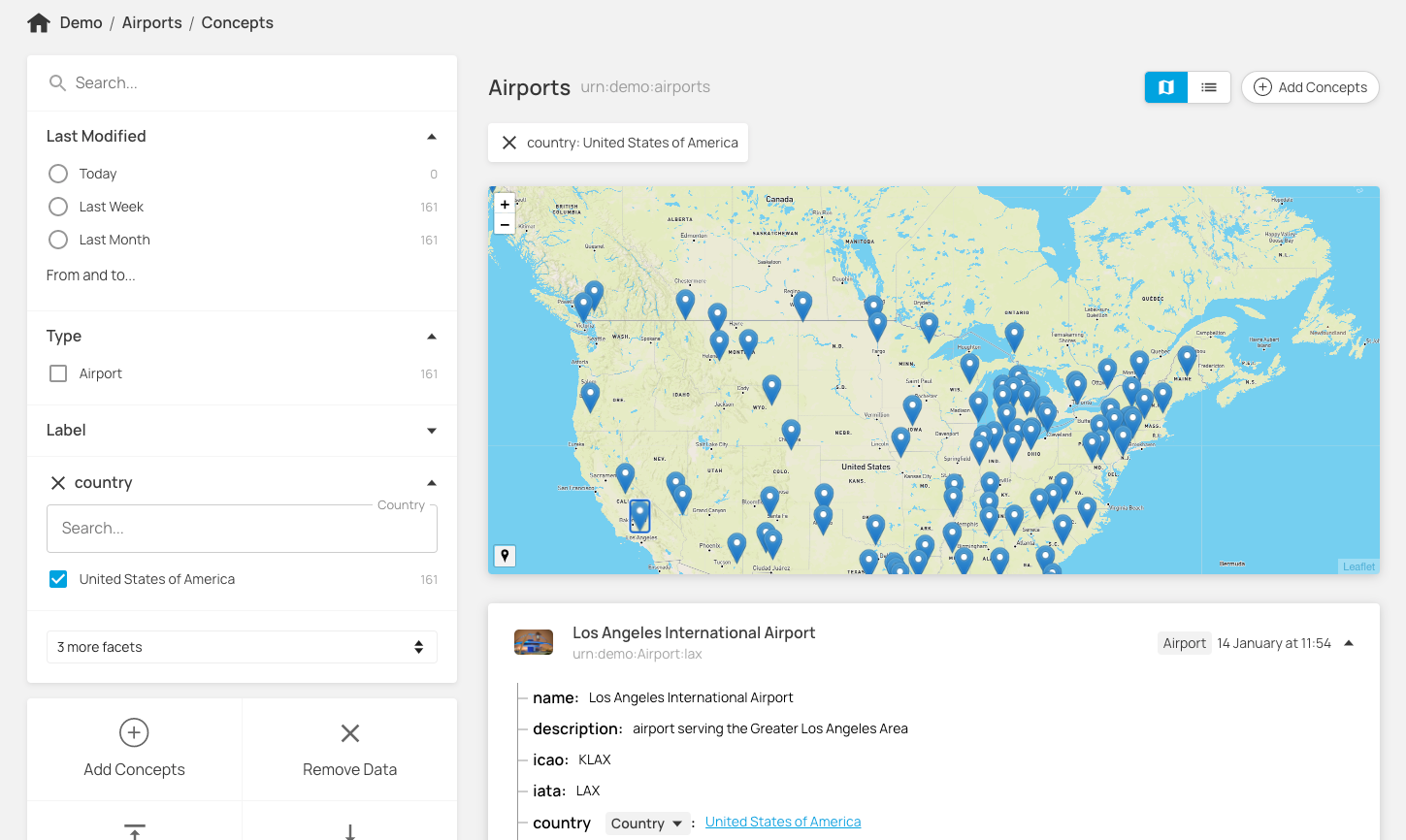Here is a detailed and cleaned-up descriptive caption for the image:

---

The screenshot showcases a web page with a subtle, pale gray background. The layout features several white rectangular sections. On the left side, there are vertically oriented white rectangles, while on the right side, the rectangles are horizontally oriented. Notably, the top right section stands out with a bright sky blue background, representing water, overlaid with a map of the United States and parts of Canada. This map truncates the southern portion of the U.S., excluding Mexico, and is populated with inverted blue teardrop location markers, each featuring a white dot at their center. These markers denote airports.

At the very top of the image, a navigation path reads "demo/airports/concepts.” Just below, within a vertically oriented white rectangle, there is a search bar, followed by "Last Modified" with selectable radio buttons for "Today," "Last Week," "Last Month," and a date range "From" and "To" fields. Under this, a "Type" section includes an unchecked checkbox labeled "Airport." Further down, another search bar lets users enter a country, defaulting to the "United States of America," which appears as a checked checkbox.

Lower in the same section, the top portion of another text box is visible, featuring a circled plus sign labeled "Add Concepts" and an 'X' icon labeled "Remove Data," suggesting further options lie below.

To the right, on the map, there are zoom controls with plus and minus signs typical of interactive maps. Below the map, under the label "Airports," is another search bar with an 'X' icon, displaying "Country: United States of America," indicating that users can search for and replace this entry.

A clicked blue location marker on the map is highlighted with a thin outline, revealing a pop-up containing details about Los Angeles International Airport (LAX), including its name, description, icon, IATA code, country, and county, among other attributes.

---

This caption thoroughly describes the elements and layout of the web page screenshot while including relevant details about the interactivity and content displayed.